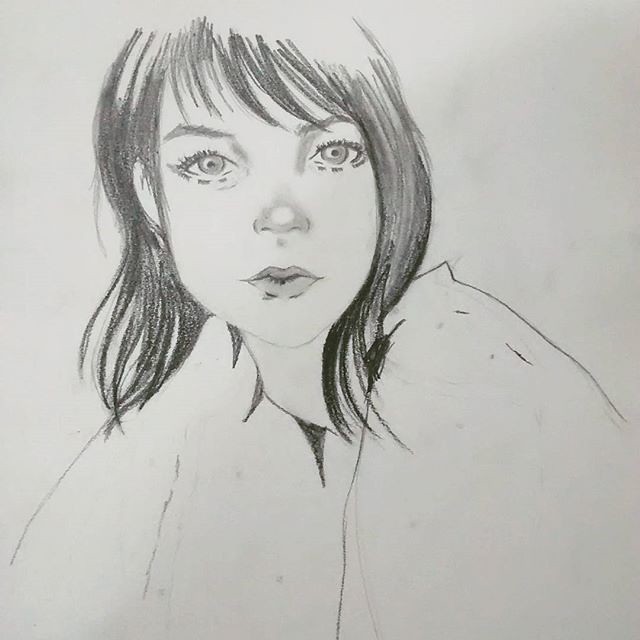A meticulously detailed charcoal sketch portrays a young girl with captivating, light-colored eyes—possibly blue or green—gazing directly into the viewer's perspective. Her delicate button nose, noticeably shaded for emphasis, and her subtly parted lips evoke a sense of innocence and curiosity. Her dark, shoulder-length hair frames her face softly, complementing her contemplative expression. Her right hand rests gently below her neck, adding an element of introspection to the composition. She is adorned in a nondescript blouse which ambiguously suggests the presence of a coat or similar garment, the folds and shapes blending seamlessly with the artistic strokes. The sketch showcases her serene yet enigmatic aura, highlighted by the precise use of charcoal pencils, offering a testament to the artist's skill in capturing both detail and emotion.